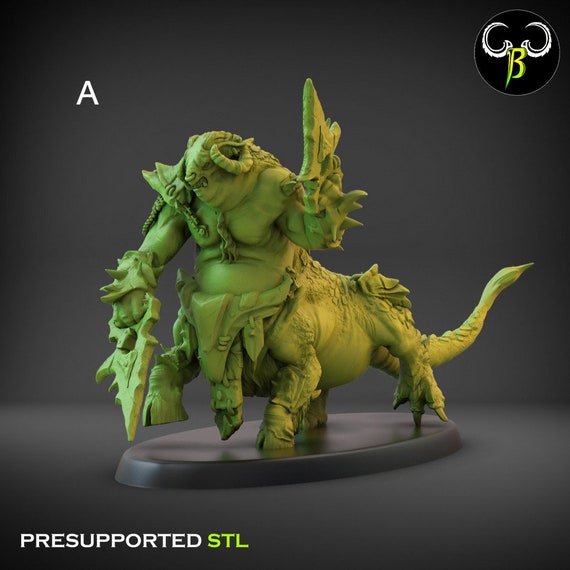The image depicts a detailed, green, 3D model of a fantastical creature, set against a dark black and gray background. The creature, which appears to be designed for 3D printing, is labeled "pre-supported STL" in the bottom left corner (with "pre-supported" in white and "STL" in green). The upper left corner of the image features the letter "A," while the upper right corner shows a logo with a green letter "B" adorned with horns. 

The creature itself is a hybrid beast with a blend of anatomical features. It has four legs: the front ones are hooved like a cow, while the back ones have sharp claws reminiscent of a dragon's. Its tail is long and sharp, adding to its menacing appearance. The body of the creature is robust and muscular, yet chubby in nature. Its face resembles that of a cow or some beast, complete with curling horns on top. Notably, its arms are more humanoid, ending in fists that grasp two blades. The intricate design also features additional arms akin to those of a grasshopper and overall, the creature is covered with various protrusions and detailed parts, emphasizing its complex structure.